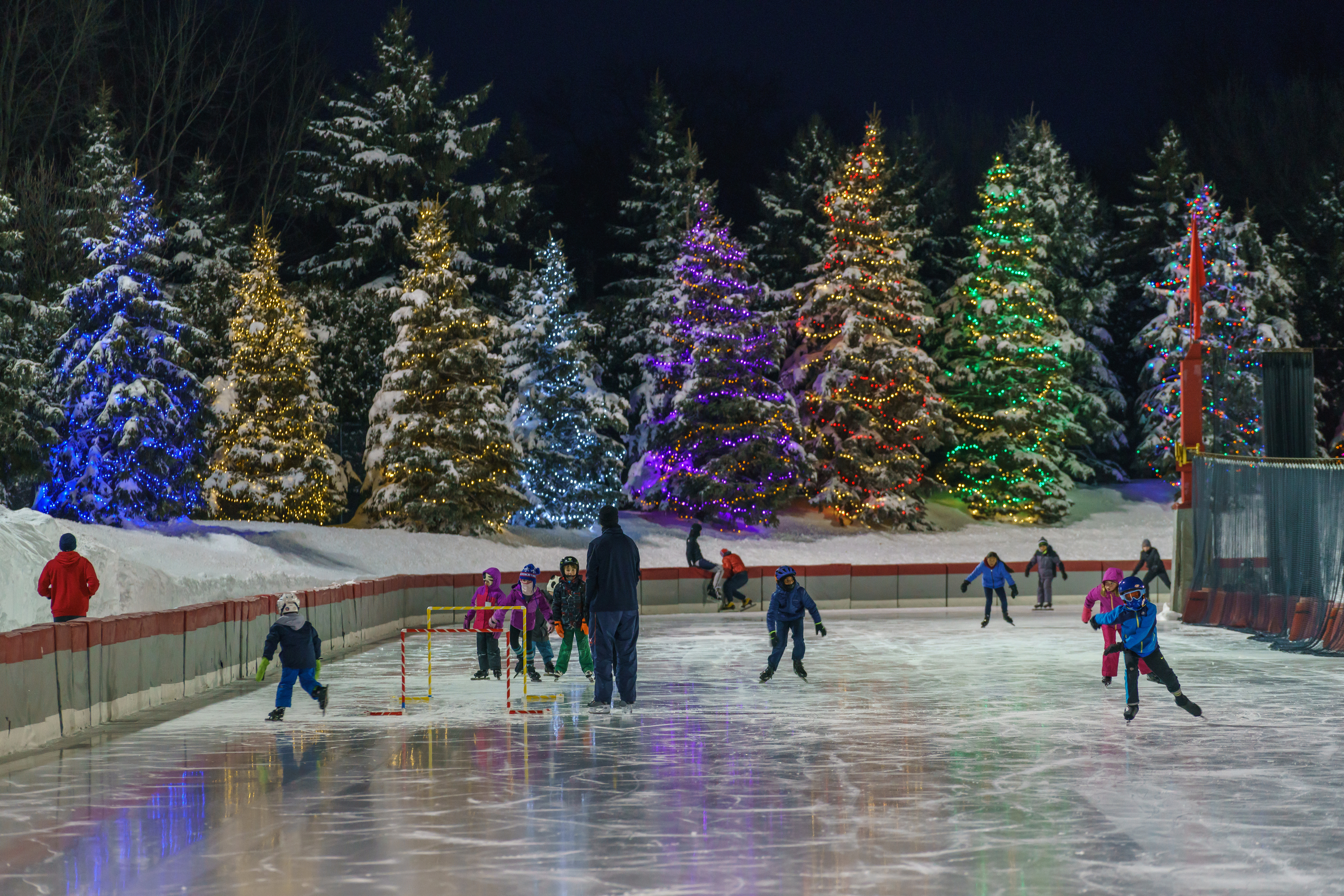The image depicts a lively outdoor ice skating rink at night during the Christmas season. The scene is illuminated by an array of beautifully decorated evergreen trees in the background, each adorned with colorful Christmas lights in shades of blue, aqua, purple, gold, and green, some blanketed with a light layer of snow. In the forefront, the rink is bustling with activity: several children in various colorful jackets—blue, red, and pink—are skating towards the viewer, while in the middle, a man in a red jacket appears to be instructing or engaging with the group near an ice hockey goal. An adult is also seen walking along the left side of the rink. The rink is bordered by a gray, white, and red wall, and to the right, there is a fenced-off section, adding to the festive and organized atmosphere. Snow covers the ground, enhancing the wintry charm of this holiday scene.